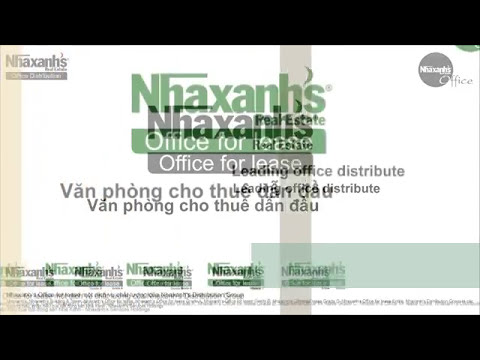The advertisement graphic prominently features a non-English (likely Vietnamese) text, centered on a clean white background. It includes black banner lines at both the top and bottom, with a very pale yellow line on the far left and a tan line in the center, both extending vertically. At the top, within the white area, “N-H-A-X-A-N-H’s™” is written in green letters, accompanied by a smaller, gray repetition of the same text directly below. Beneath this, a green banner reads "Office for Lease," followed by a gray banner with the identical text. Below these banners, there are two additional lines of text in the foreign language. The very bottom area of the advertisement features overlapping text, predominantly gray with some green, which is difficult to decipher.